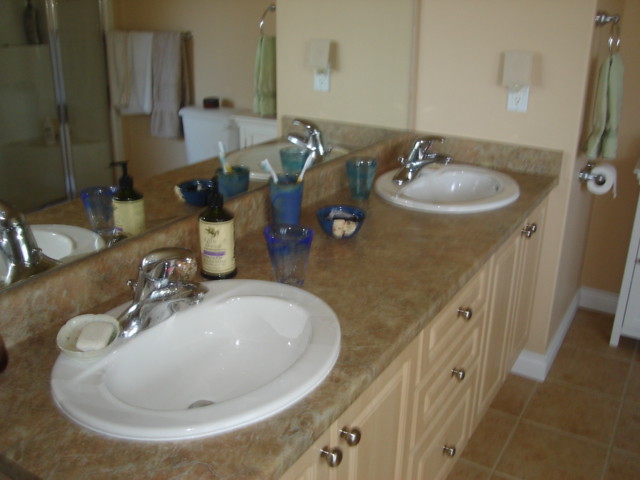The image showcases an elegant double bathroom sink setup, viewed diagonally from behind the left sink. The sinks are white and set within a marble-textured countertop with a brownish hue. A long, expansive mirror spans the wall above the sinks, reflecting the setup and giving depth to the space.

The left sink features a soap dish holding a bar of soap. Just right of this sink, a bottle of hand soap and a stylish blue glass are neatly placed. Centrally positioned between the two sinks, a cup holds two toothbrushes, accompanied by a small bowl containing an unidentified object. 

The right sink mirrors the left in its simplicity, with another matching blue glass placed to its left. Beneath each sink are tan-colored cupboards with chrome knobs that open outward, offering storage space. Three drawers are centrally located between the cupboards under the sinks, providing additional functionality.

A light switch or outlet is visible on the wall at the end of the counter. To the right, the space curves around a corner, where a roll of toilet paper and a neatly hung towel can be seen, adding to the practicality and complete functionality of the bathroom's design.